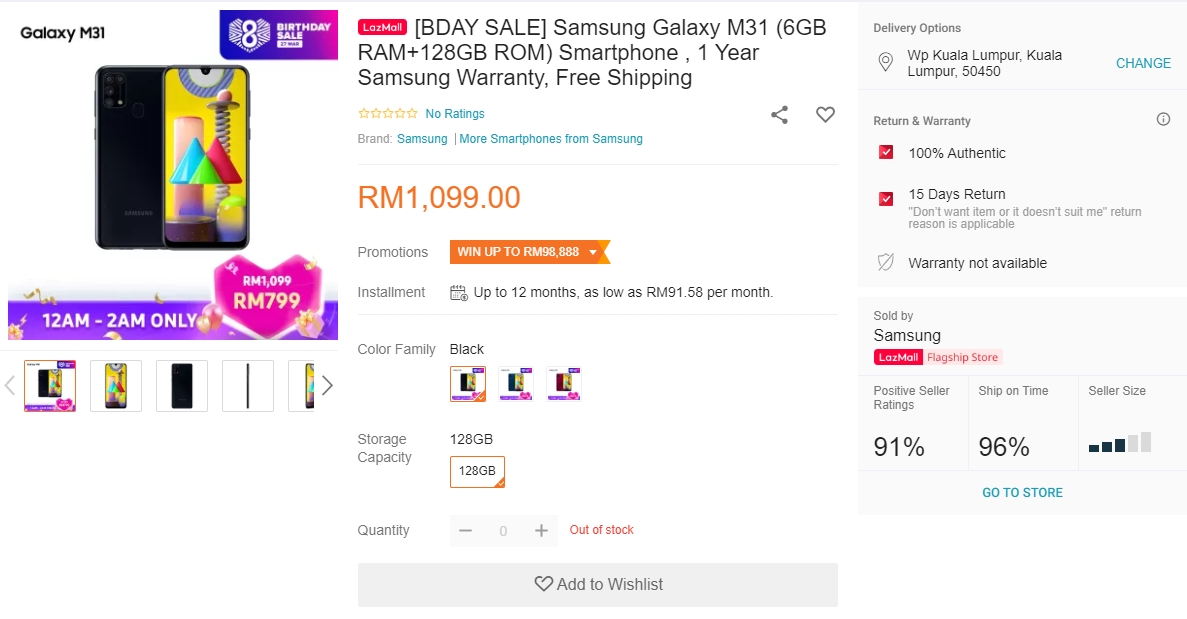The image depicts a product purchasing page for a Samsung Galaxy M31 smartphone. On the left side of the page, "Galaxy M31" is prominently displayed in black text above a stock photo of the smartphone. The phone's illuminated screen features a yellow background adorned with colorful shapes, including three triangles—one large blue, one smaller green, and another large red triangle. Beneath the main image, there are smaller preview images showing the phone from various angles and in different power states.

Centered on the page, a promotional banner announces a "Birthday Sale" for the Samsung Galaxy M31, which boasts 6 GB of RAM and 128 GB of ROM. The phone comes with a one-year Samsung warranty and the offer includes free shipping. Just below, a section for ratings is shown, displaying several stars that are not filled in, accompanied by the text "No ratings" in blue.

The product is listed with a price of RM 1,099, highlighted in orange. On the far right, additional information is presented in a light gray rectangular section, including details about delivery options, returns, and warranty. The page claims the product is 100% authentic and offers a 15-day return policy.